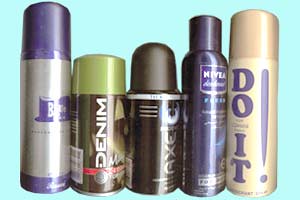This image showcases a series of five personal care products, predominantly spray cans, neatly lined up against a light blue, featureless background which adds no additional context. From left to right:

1. The first canister is tall and cylindrical with a metallic body adorned with purple accents, and it has a matching purple cap.
2. Next is a shorter canister labeled "denim." It features a green lid and displays the word vertically. The body of this can is a mix of pale dark green hues, with additional graphic designs.
3. The center canister is a black aluminum spray can for Axe deodorant, with a uniform black top slightly smaller in diameter than the can itself.
4. Following that is a Nivea product, almost as tall as the first can, characterized by its blue color and blue cap, again slightly narrower than the main body.
5. The final canister is beige with a matching beige cap. It features "do it" written in purple vertically along with an exclamation mark running the length of the can.

Each product features distinct colors and designs, emphasizing their individual branding.